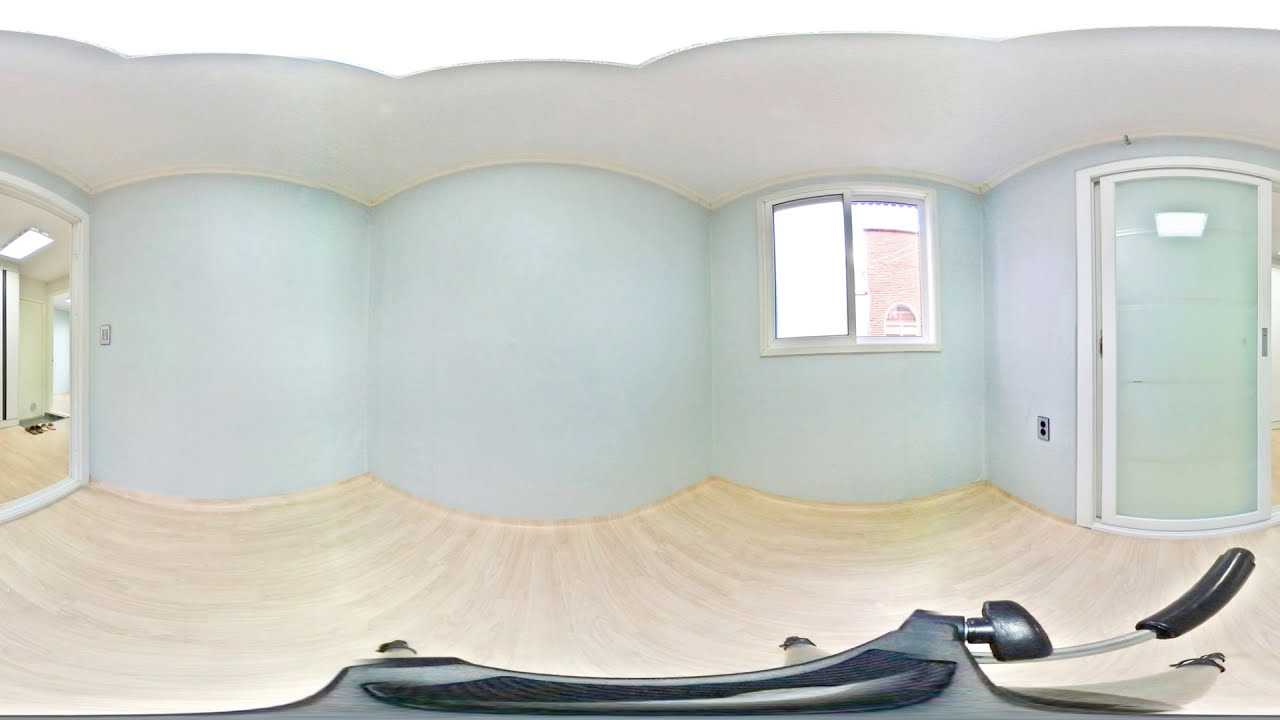The image depicts an indoor room with distinctive, cartoonish characteristics. The room features a white ceiling and pine-colored hardwood floors that appear completely clean. The walls are painted in a light green or teal hue. The room is designed with a series of curved, convex walls that seem to bulge outward, creating a somewhat distorted and unrealistic appearance. 

At the center of the background wall, there is a window that allows daylight to flood the room, flanked by a door to the left and another to the right. Each door matches the wall color, maintaining the light green or teal theme. The right door appears to lead to another room, while the left door is closed. 

On the left side of the image, there's an item that is difficult to identify but resembles parts of a bench or a table, placed on the floor. To the left, there is a mirror framed in detailed white wood, which reflects a part of the adjacent room. The main focus remains on this empty room that has minimal decor and no occupants, emphasizing its spacious, uncluttered nature.